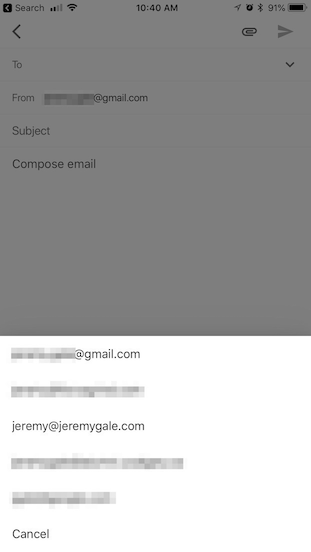The image appears to be a screenshot taken from a cell phone, showcasing an email composition screen within a Gmail app. 

At the top left of the screen, there is a small black square with a white arrow pointing left, next to the word "Search." Adjacent to these icons, signal indicators and a Wi-Fi signal icon are visible, implying a connected status. The time displayed in the center of the status bar shows 10:40 AM. 

On the top right, several icons are present: an unspecified icon that might relate to privacy or location settings, an alarm clock icon, and a battery icon indicating a 91% charge.

Underneath the search field, there is a left-pointing arrow icon. To the far right, a paper clip icon represents attachment options, next to a gray right-pointing arrow. 

In the email body, there is a dropdown menu showing two-character space. The subsequent lines read as follows: "From" followed by an obscured email address ending in "@gmail.com"; "Subject"; and "Compose Email." All these details appear grayed out against a black background.

Towards the bottom part of the screenshot, the background shifts to white, displaying several previously used Gmail accounts, which are largely obscured except for the domain "@gmail.com". One visible email address is "jeremy@jeremygale.com", while other details are blurred or scratched out.

At the very bottom of the screen, the word "Cancel" is clearly displayed.